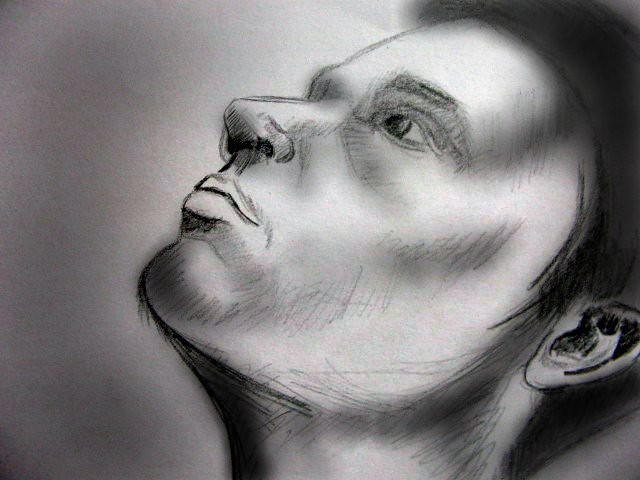This detailed sketch, likely created with heavy black drawing charcoal or pencil on black paper, portrays a figure with ambiguous ethnicity, possibly male, shown from the neck up. The head is tilted back and oriented towards the upper left corner of the image, while the eyes gaze upwards. Short dark hair frames the serious, tension-filled face that features high cheekbones and a straight, small nose. The sketch makes extensive use of grayscale shading and shadowing, especially around the chin, neck, and ears, highlighting the detailed craftsmanship. The face spans from just left of the center to the top right of the composition, with the jawline strongly defined by black strokes, giving the piece a realistic and carefully proportioned appearance, reminiscent of a high-level art student's work.